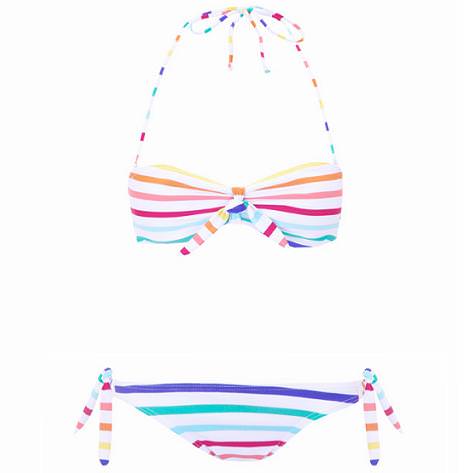The image depicts a two-piece bikini set against a completely white background, which enhances the vibrant colors of the swimwear and suggests a studio or digitally manipulated setting. The bikini features a cheerful, multi-colored stripe pattern reminiscent of a candy cane but with a bright and varied palette that includes teals, baby blues, bright pinks, light pinks, oranges, yellows, magentas, and whites. The bikini top occupies the top half of the image and is designed with a bow tied at the center and straps that come down to support the bust. It ties around the neck, with some versions mentioning small bows on the straps. The bottom half of the image displays the bikini bottoms, which share the same colorful stripe pattern. These bottoms are adorned with small bows on each side of the hips, accentuating the playful and vibrant design. The colors on the top and bottom appear to complement and mirror each other, though one version describes a subtle reversal in the color order between the two pieces.